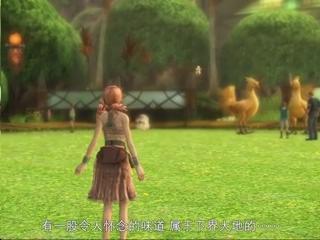The image appears to be a rendered scene, likely sourced from a video game. In the foreground, we see the back of a woman standing with her arms slightly raised and positioned behind her. She is wearing a brown skirt and a small brown top, which may have a lighter midsection. It is unclear whether this lighter section is part of her attire or her light skin tone showing through. She has light-colored hair that cascades down her back.

The background reveals a lush field of green grass punctuated by a few verdant trees. Towards the horizon, a large, somewhat indistinct structure looms, marked by columns and archways, but the details are blurred and hard to discern. Off to the left in the distance are several yellow, chicken-like birds that stand taller than nearby human figures. These birds, although avian in shape, tower over the humans, adding a fantastical element to the scene. At the bottom of the image, a stamp of white characters in an unreadable language is visible, likely indicating in-game text or a watermark.